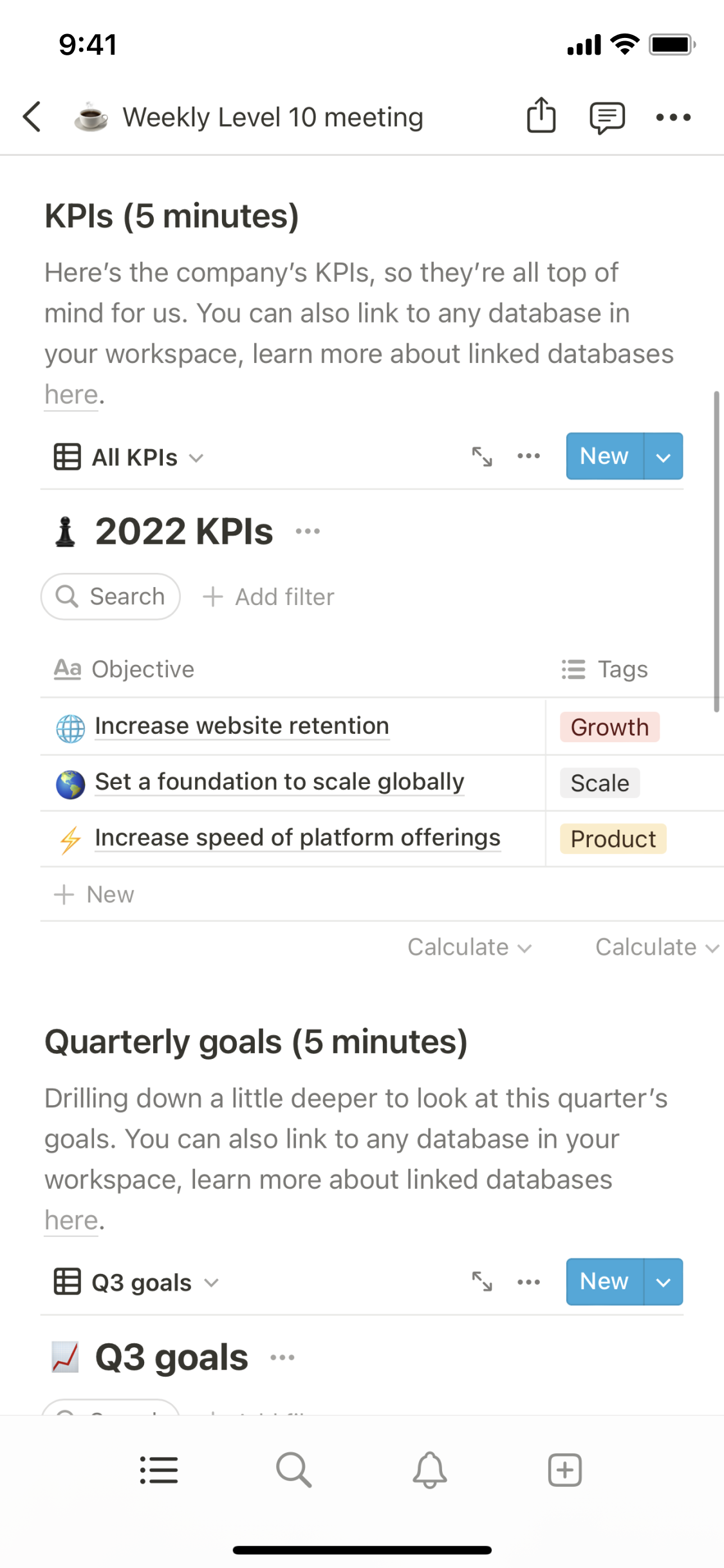This image is a detailed screenshot of a digital workspace interface, potentially from a project management or organizational tool. It captures various elements and sections designed for team collaboration and task management.

At the top of the image, the header displays crucial status icons: the time "9:41," a Wi-Fi symbol indicating connectivity, and a battery icon showing power status. Below that, titled in bold black font, is "Weekly Level 10 Meeting," accompanied by a white coffee cup icon and a back arrow that likely navigates to a previous page.

The central part of the screenshot is occupied by a section titled "KPIs - 5 Minutes" in black text, where the company’s Key Performance Indicators (KPIs) are listed to keep them top of mind. A message suggests linking to any database in the workspace and offers additional information about linked databases. The section is collapsible, as indicated by a downward arrow. Users can interact with elements like a gray arrow, three options represented by dots, and a blue and white "New" button.

Listed KPIs include:

1. **Increase Website Retention**: Marked with a blue globe icon and tagged "Growth" in red text.
2. **Set a Foundation to Scale Globally**: Paired with a green and blue globe icon and tagged "Scale" in gray.
3. **Increase Speed of Platform Offerings**: Denoted by an orange and black lightning bolt icon and tagged "Product" in orange.

There's an option to add new KPIs, signified by a gray "New" button with a plus sign.

The next section, titled "Quarterly Goals - 5 Minutes", provides an in-depth look at the current quarter's objectives. It repeats a prompt about linking to databases and offers further details on linked databases. Listed goals under "Q3 Goals" include a similar interactive arrow and dot elements, along with a "New" entry button.

At the bottom of the screenshot, there's a user interface or toolbar featuring icons: a gray magnifying glass (search), a gray bell (notifications), a gray square, and a black line, representing various functions or navigation shortcuts within the tool.

Overall, the screenshot is a comprehensive view of a structured meeting agenda and task tracking, facilitating organized and efficient team collaboration.